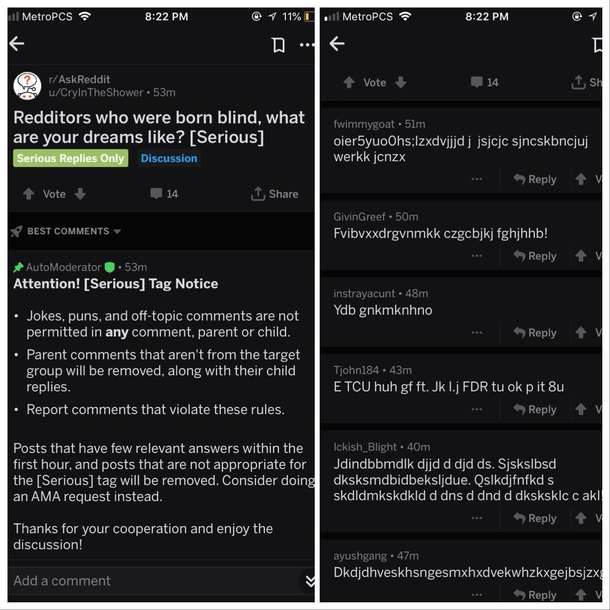This composite image consists of two screenshots taken from a mobile phone at 8:22 p.m., with the device set to dark mode, resulting in a black background. The screenshots showcase a Reddit page from the subreddit r/AskReddit. The post in focus, created by the user "u/cry_in_the_shower" 53 minutes prior, is titled "Redditors who were born blind, what are your dreams like?" with a "SERIOUS" tag denoted in brackets to emphasize that only genuine replies are sought. Below the post, is a green rectangle stating "Serious replies only" and a purple-colored label tagged "Discussion". 

The initial comment displayed is from AutoModerator, outlining the etiquette expected in the thread: "Attention! Serious Tag Notice: Jokes, puns, and off-topic comments are not permitted in any comment—parent or child. Parent comments that aren't from the target group will be removed along with their child replies. Report comments that violate the rules."

However, the subsequent comments displayed in the screenshots veer away from the intended seriousness. They are filled with offensive and nonsensical remarks, mocking the query by sharing irrelevant text and gibberish, making insensitive jokes about the inability of blind individuals to read or type.